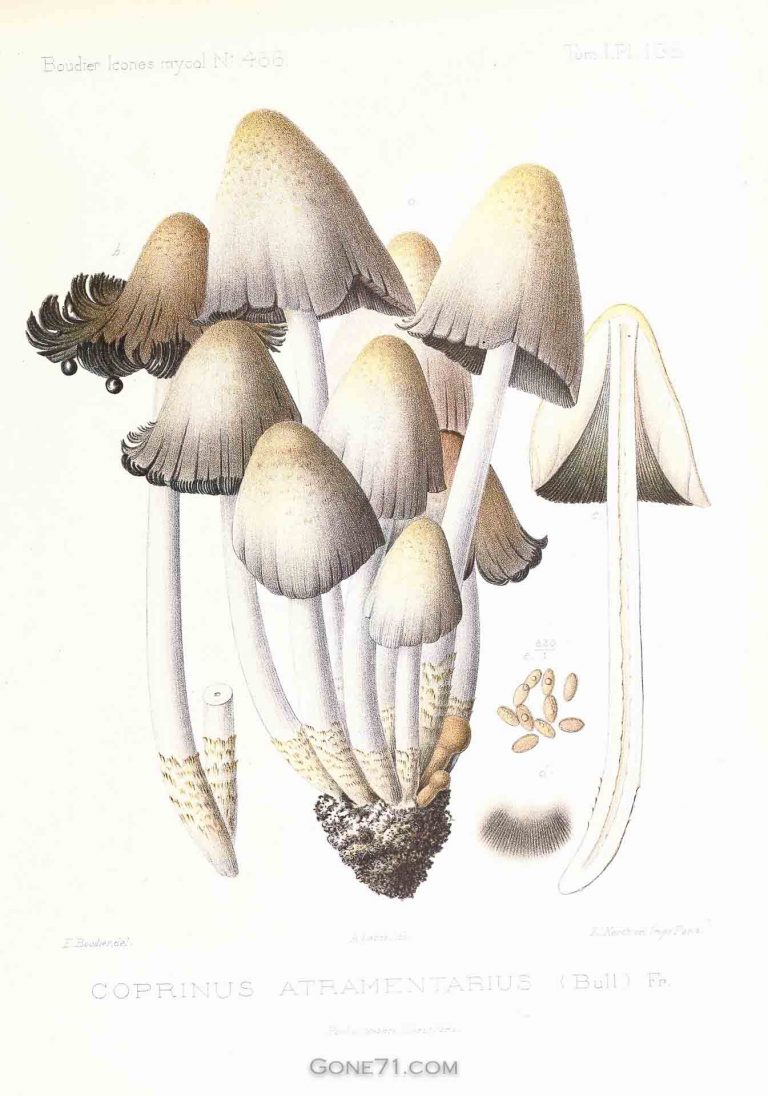This image from gone71.com features an intricately detailed drawing of various tall mushrooms. The artwork, set against a white background with a faint beige hue, showcases around a dozen mushrooms of different shades of white, tan, and brown. Most of these mushrooms share a common triangular black base, resembling soil, while two mushrooms stand independently off to the sides. Between the central cluster and the rightmost mushroom are several oval cream-colored cells, with thin, faint lines below them that suggest a caterpillar-like pattern. Various texts adorn the image: the top left corner ambiguously reads "Boulder Icones," while the top right corner contains hard-to-read text. At the bottom, in clearer writing, it states "Coprinus Atramentarius" alongside the website watermark "gone71.com." This visually compelling drawing emphasizes the diverse and textured appearance of the depicted mushrooms.